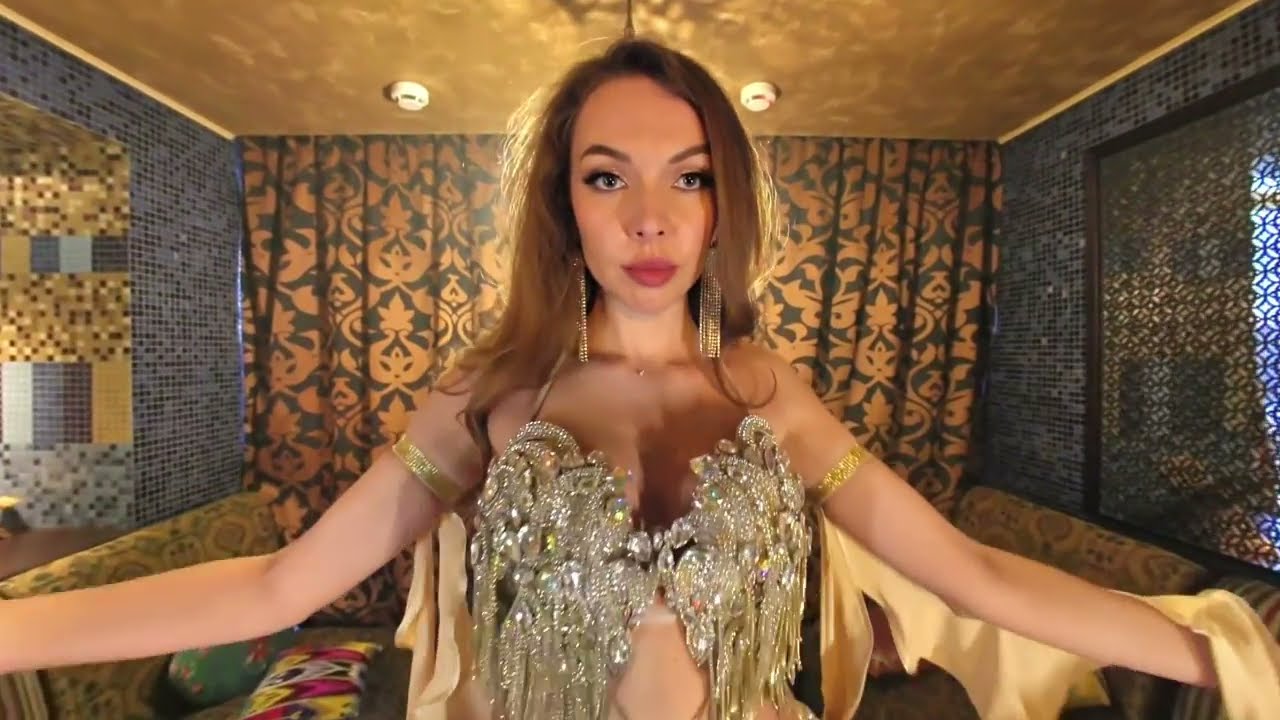In the photograph, a young woman of possibly Caucasian or mixed ethnicity with fair skin and slightly fluffy, light brown or dark blonde hair is facing the camera from about the torso up. She wears heavy makeup with large eyelashes and pink or red lips. Her attire is striking, featuring an elaborate bustier top adorned with gold, silver, and gem-like sparkles arranged to resemble wings, leaving her midriff exposed. Long, dangling earrings that glint gold or silver dangle from her ears, and her upper arms are adorned with golden bangles. A golden silk cloth or a yellow cape drapes over her left arm, which is extended out to the side, mirroring her similarly positioned right arm.

The setting is an intriguing, small indoor room where the ceiling is gold-colored. The back wall is covered by a curtain with a blue background featuring gold stars and leaves or a floral design. The left and right walls are adorned with blue tile and feature a variety of colorful seating areas. The right side of the room also has a screened-in portion, allowing a view outside, while the left side includes a mirror that adds depth to the space. The overall effect is one of intricate and vibrant detail, complementing the woman's elaborate outfit.